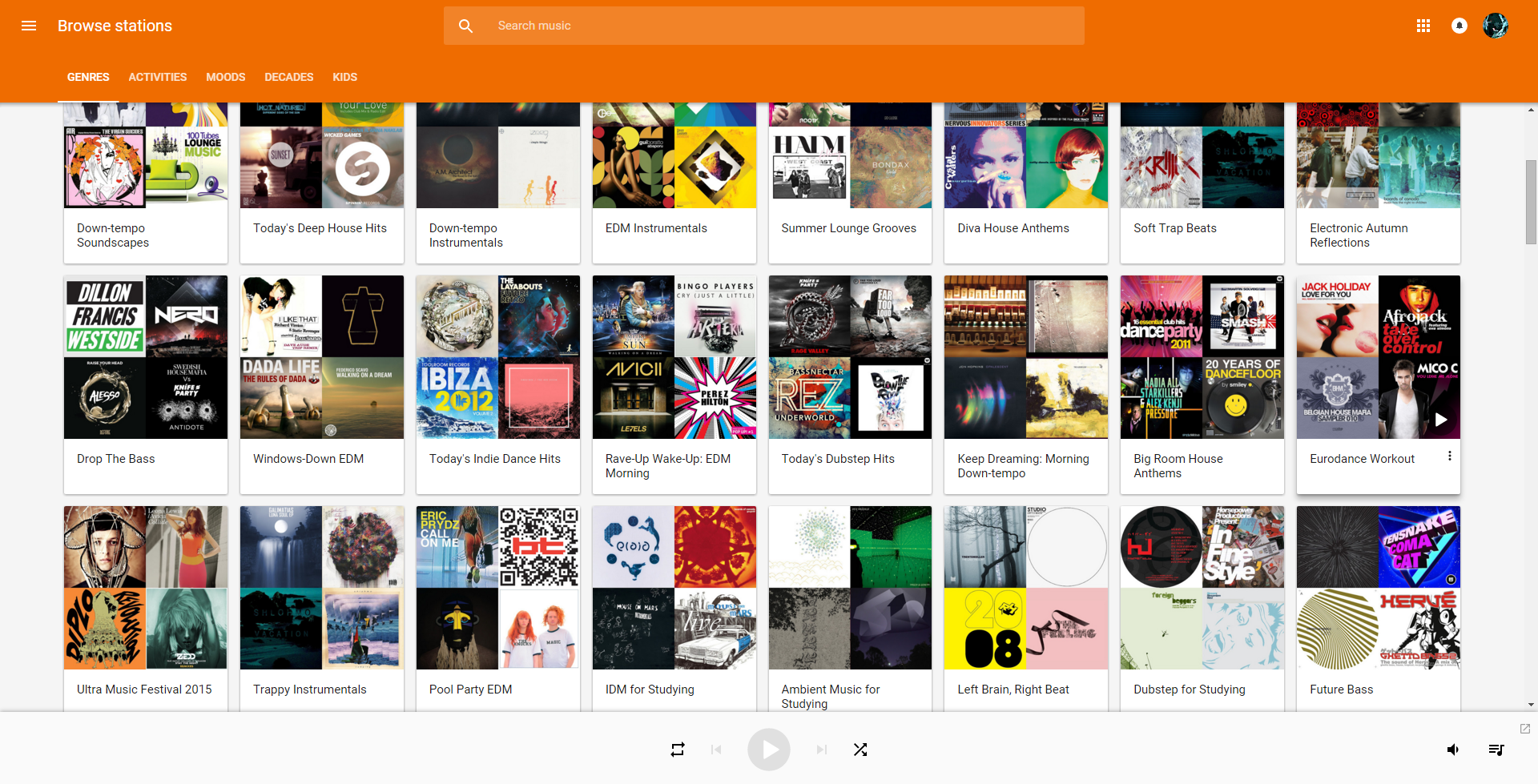This image captures a computer screen displaying a music streaming website, specifically the "Browse Stations" section. At the top of the webpage, there's an orange rectangular header featuring white text. On the far left of this header, three horizontal lines are visible, indicative of a menu icon. Beside it, the text reads "Browse Stations." Further to the right, there's a brighter orange clickable rectangle labeled "Search Music," accompanied by a white magnifying glass icon.

Just below this main header, still within the orange section, there are clickable categories labeled "Genres," "Activities," "Moods," "Decades," and "Kids." Below these categories, the screen reveals various clickable music genres and playlists such as "Down-Tempo Soundscapes," "Today's Deep House Hits," "Down-Tempo Instruments," "EDM Instrumentals," "Summer Lounge Grooves," "Diva House Anthems," "Soft Trap Beats," and "Electronic Autumn Reflections." These titles are organized in a top row, followed by a middle and a bottom row, each containing an array of music options to explore.